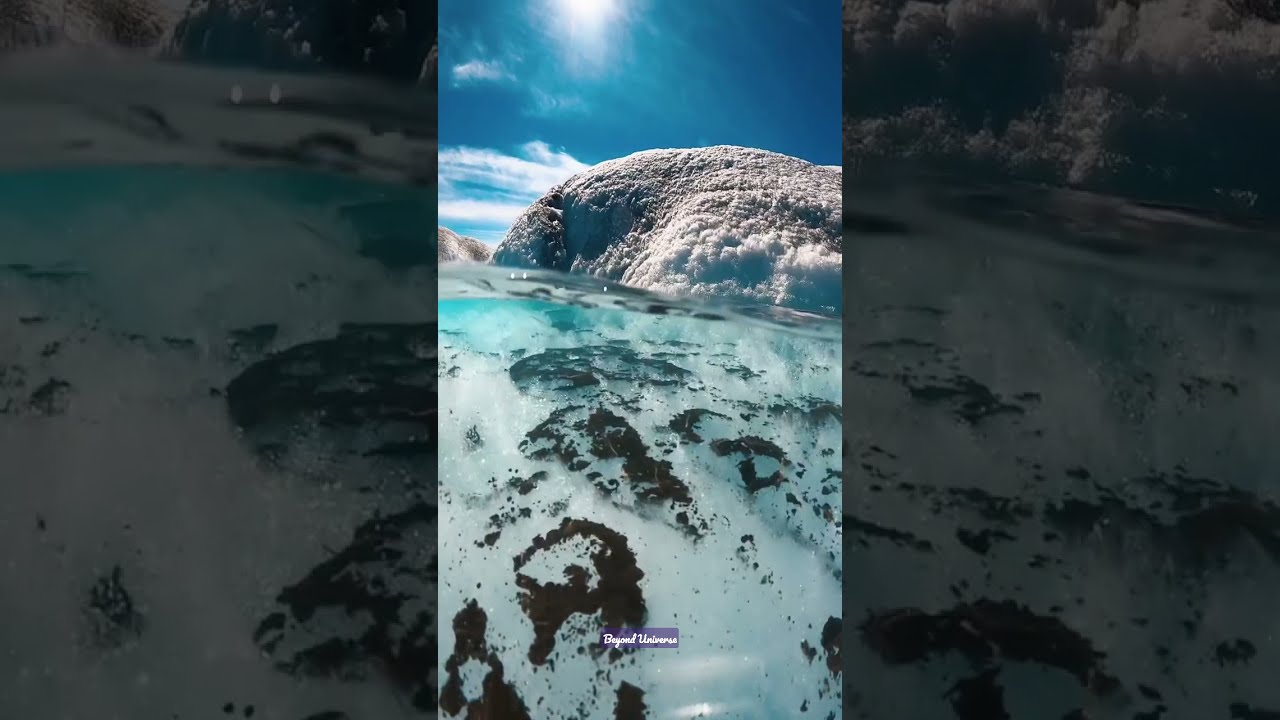The image depicts a serene seascape with a large, rounded iceberg or snowy rock formation at the center, partially submerged in crystal-clear, bright blue ocean water. Above the horizon, a radiant sun shines brightly in a vivid blue sky that holds a few distant clouds. In the depths of the transparent water, which is shallow enough to reveal the bottom, patches of dark debris, possibly dirt or coral, are visible. The photograph is framed by two vertical sections on either side, showing zoomed-in versions of the central image, which are dimly lit, accentuating the intricate details of the iceberg and the surrounding water. At the bottom of the central image, the phrase "Beyond the Universe" is prominently displayed in a purple rectangle in white text.